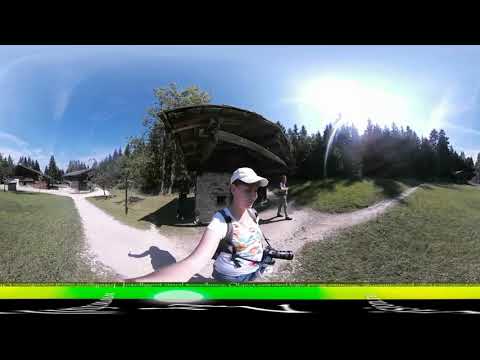A woman in a white cap and white shirt with hints of orange and green stands at the center of the image, slightly lower in the frame. She is taking a selfie with her phone in one hand, while a DSLR camera hangs from a strap around her neck. Behind her is a brown and tan sheltered building. To her right, a walking path of light tan gravel meanders through the landscape, bordered by light green grass and dark green trees. The path extends leftward, leading to additional distant structures. The sky above is a mix of light blue with white, partly cloudy areas, adding a serene backdrop to this wide-shot, somewhat distorted park scene.